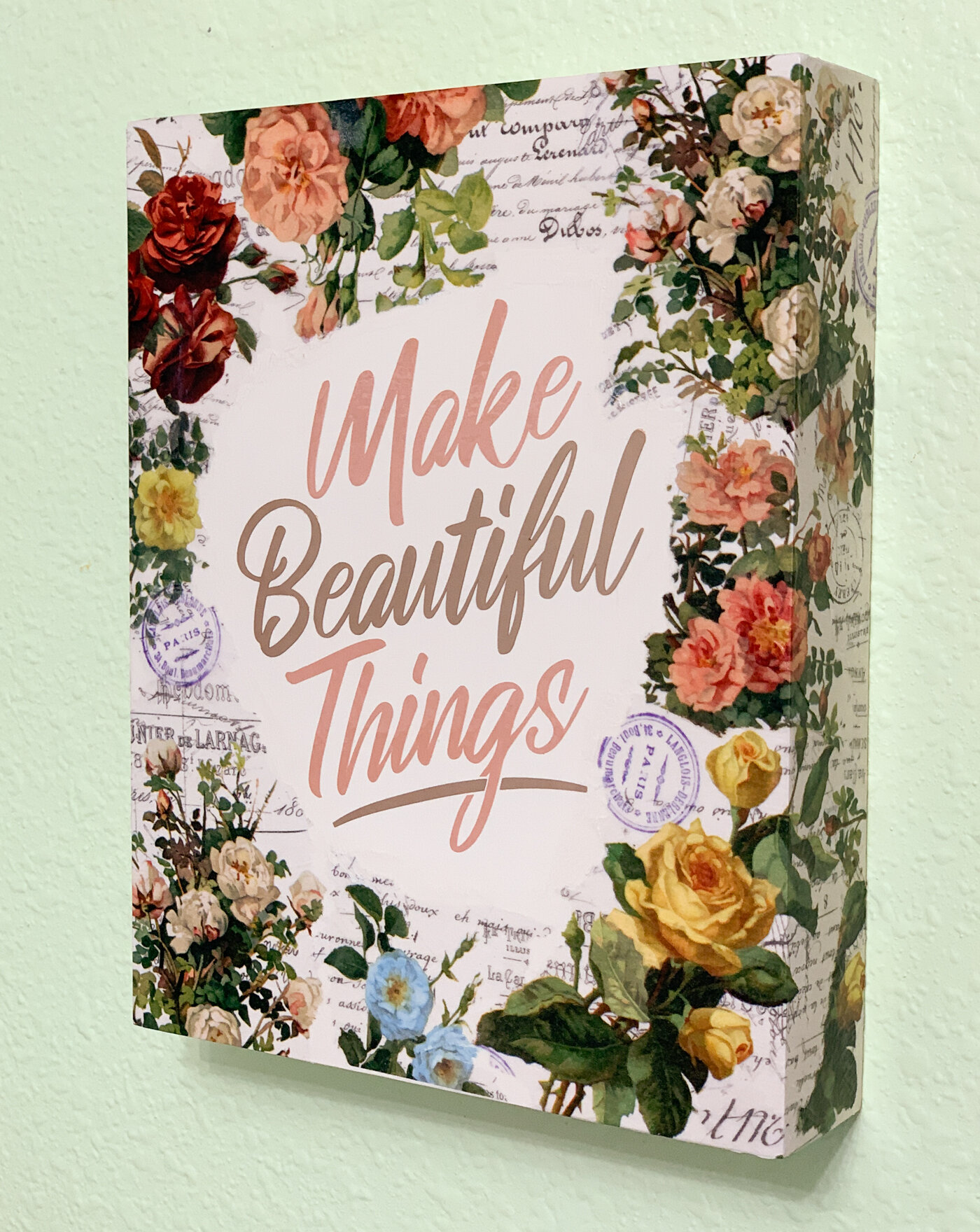The image is a rectangular wall hanging printed on cloth or canvas, wrapped around a thick wooden frame, about one and a half to two inches deep, adding a three-dimensional effect. The design extends onto the sides and top of the frame, enhancing its aesthetic appeal. The central focus is the elegantly written cursive text that reads "Make Beautiful Things," surrounded by a lush halo of various flowers, including yellow roses, pink zinnias, and possibly marigolds. There are also hints of other flowers in white, blue, and red hues, complemented by green leaves. Interspersed within the floral arrangement are rubber stamp images, including distinct ones that reference Paris, giving it a whimsical travel-themed touch. There is also some cursive handwritten text in the background, mostly obscured by the flowers. The overall neutral tones of the text make it versatile enough to fit into any room's decor.